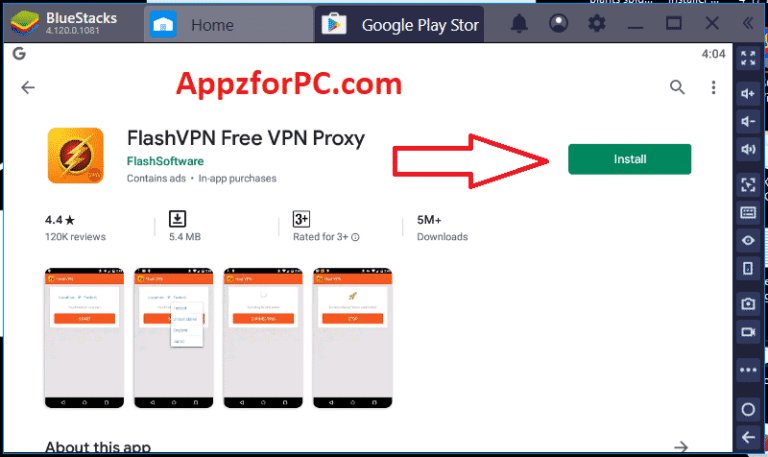The image showcases the interface of the BlueStacks software, primarily focusing on a single window that occupies most of the screen. The BlueStacks logo is situated in the top left corner, indicating that this might be an emulator rather than a standard browser. The window has multiple tabs, with "Home" and "Google Play Store" being notably visible. 

The top right corner and right sidebar are populated with various navigation icons. The main content window is displaying a section labeled "Apps for PC" from the website APAZforPC.com, but ultimately redirects to the Google Play Store. Visible on the Play Store interface is the app "Flash VPN - Free VPN Proxy," which boasts a rating of 4.4 out of 5 stars from 120,000 reviews, and a file size of 5.4 megabytes. The app has been downloaded over 5 million times. 

A prominent green "Install" button on the right side is indicated by an arrow, inviting users to download the app. Below this button, the app's preview images are displayed; there are four images in total, showing various steps in the app’s usage process, though they appear to be very similar or repetitive.